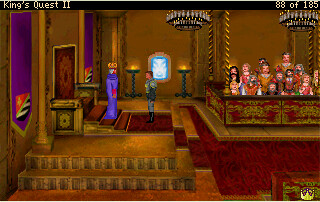This screen capture from the video game "King's Quest II" (displayed with Roman numerals in yellow text on a black bar at the top) depicts a detailed king's court scene within a castle. The upper right corner shows game progress as "88 of 185." The room features dark brown walls and deep maroon carpeting with zebra-like black designs. Central to the image, a king, distinguished by his golden crown with red accents and robes of deep purple and red, stands in front of his throne, which is positioned on a raised platform and flanked by purple banners. A knight in gray armor stands opposite the king below the steps. To the far right, a group of onlookers, possibly villagers or court members, is seated in a box-like area, attentively observing the interaction, further enriching the medieval atmosphere depicted.